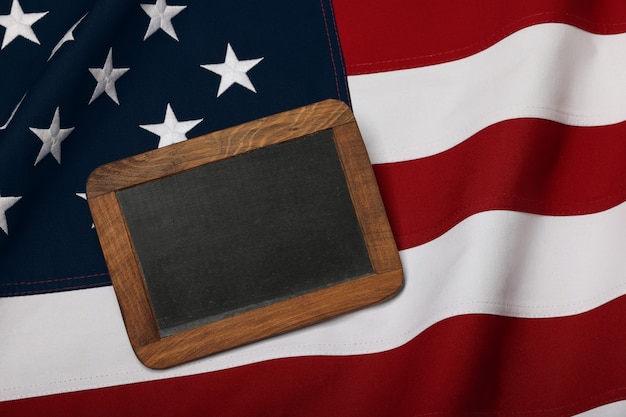This close-up image captures a detailed section of an American flag. Dominating the frame is the blue field adorned with ten visible white stars, some fully visible and others partially obscured, giving the impression of a constellation partially hidden by the night sky. The red and white stripes extend horizontally across the image, showing a gentle ripple as if caught by a light breeze. Enhancing the scene is a wooden-framed, tablet-shaped blackboard positioned atop the flag. The blackboard is blank and casts a slight shadow on the flag, adding depth to the image. The blackboard is slanted from the top right to the bottom left, and its position highlights the vibrancy of the stars and the purity of the stripes beneath it. The overall composition evokes a sense of patriotism through the flag’s timeless symbolism, subtly augmented by the contrasting texture and shadow of the wooden-framed blackboard.